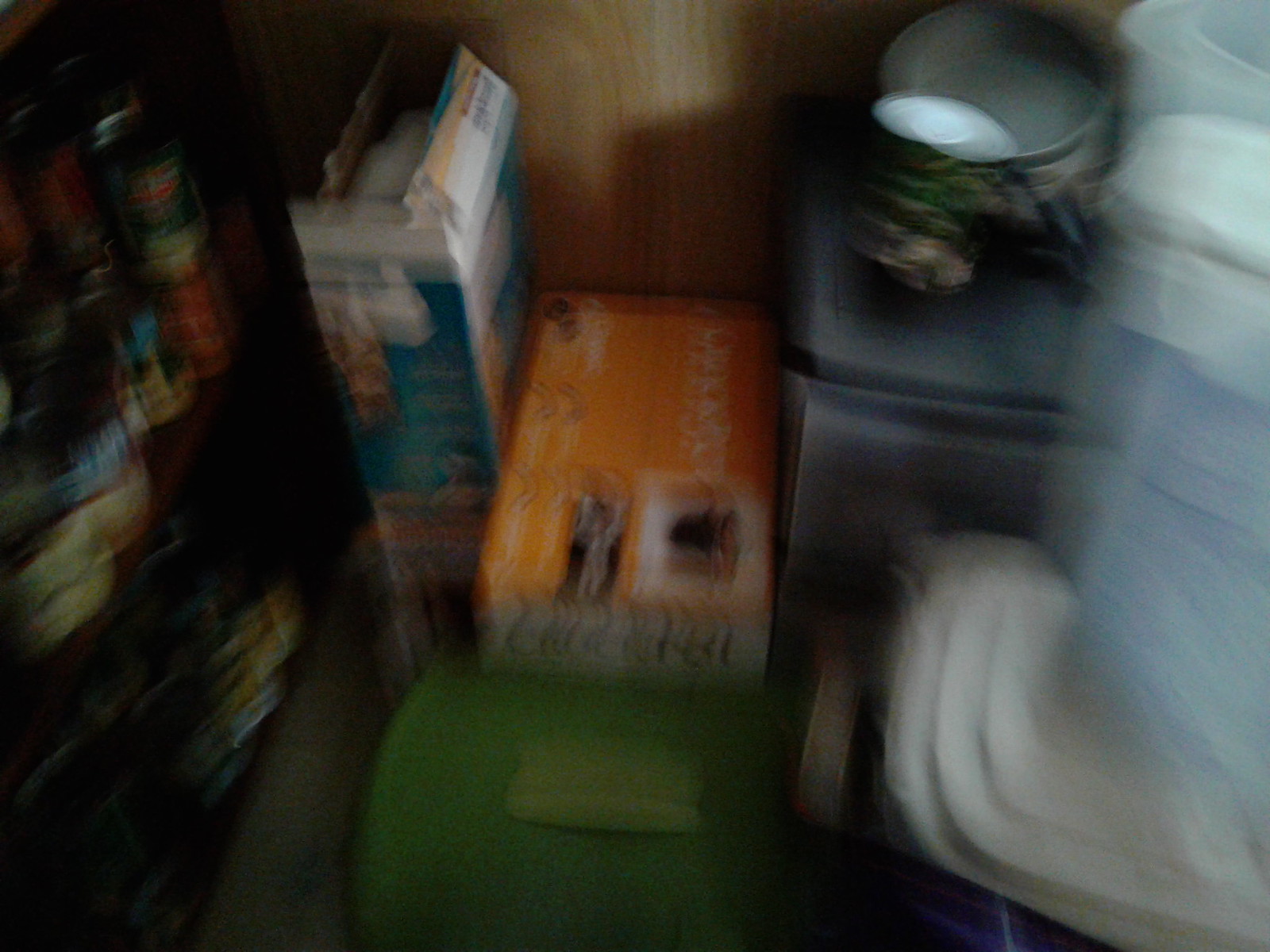The photograph showcases a cluttered storage area, captured with noticeable motion blur, likely due to the camera being bumped or moved sharply. This results in a double or triple exposure effect, creating multiple lines and distorted shapes throughout the image. In the upper right corner, several frying pans are stacked neatly, suggesting a dedicated space for kitchenware. On the left side, shelves are filled with a variety of canned goods. The lower right corner reveals a mixture of items, including an appliance and various storage containers. A chair arm is visible at the bottom center, adding to the sense of disarray. The backdrop appears to be a dark, wood-grain wall surface, contributing to the overall dim and chaotic atmosphere. Despite the blur and distortion, the image clearly depicts an area used for storing pots, pans, canned goods, and other miscellaneous items.